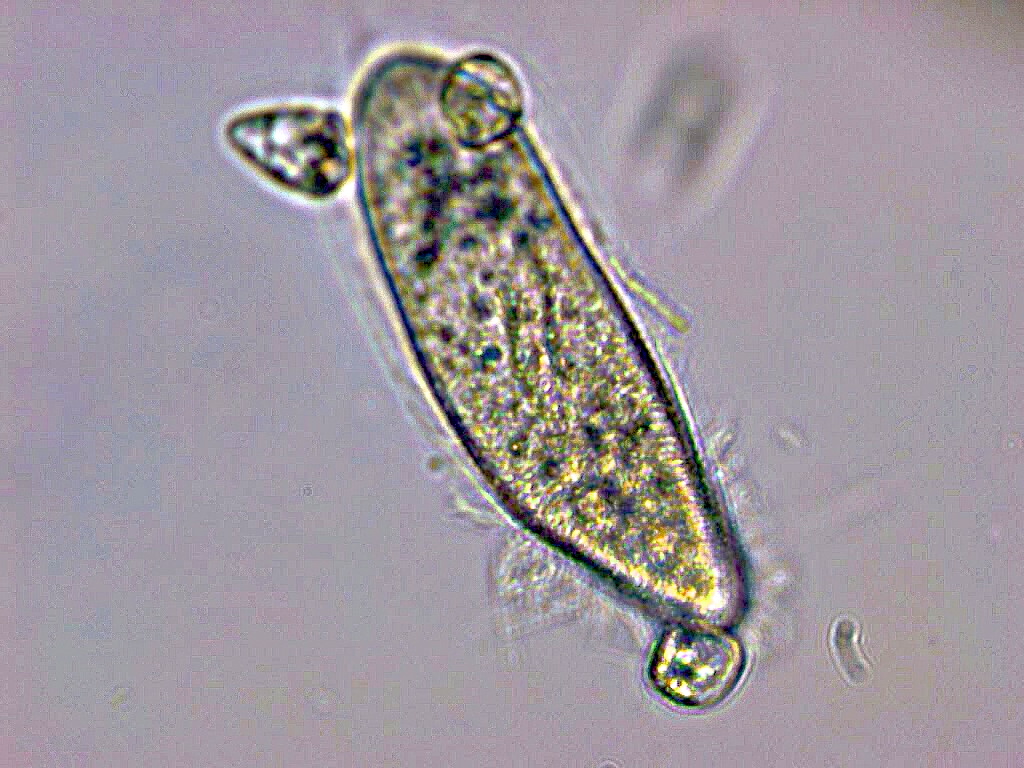This microscopy image reveals a single cell or a single-celled organism, likely a white blood cell, amoeba, or paramecium, displayed at an extreme close-up magnification. Set against a purply-blue, water-like background, the cell is oblong in shape with an oval and shimmering exterior that captures light, creating a multicolored, rainbow-like effect on its surface. The interior of the cell is kaleidoscopic, filled with various colors including greens and blues, and marked by distinct spots and lines. Notably, at the bottom of the cell is a circular, slightly square-shaped object, while near the top left lies a triangular structure, and at the top right, there is another circular element. Around the main cell are a few smaller objects, contributing to the jewel-like, sparkling appearance within the water-like environment. The overall image, despite being somewhat blurry and pixelated, captures the intricate and colorful details of the cell's structure.